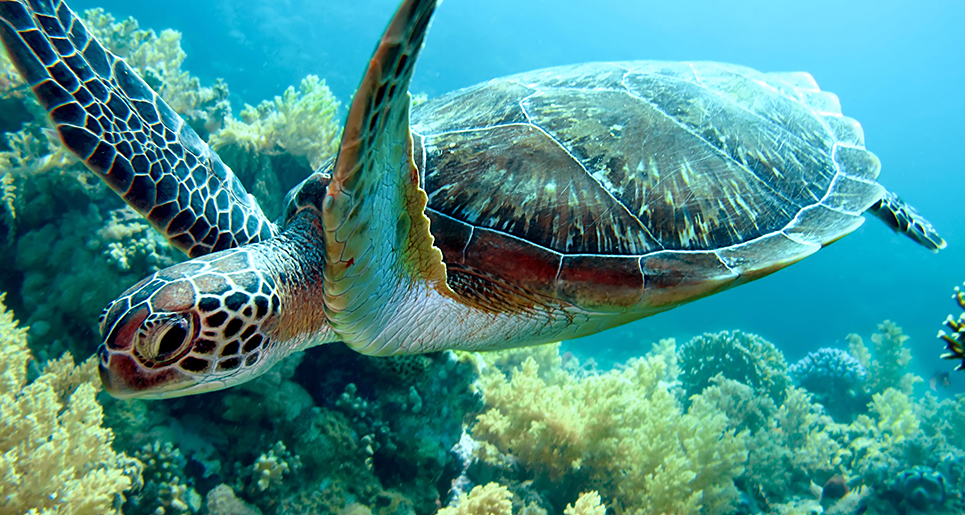This underwater photograph captures a vivid and tranquil scene of a sea turtle swimming gracefully in a tropical ocean. The close-up image focuses on the turtle's head positioned in the bottom left quadrant while its rear extends towards the top right. The turtle's front fins are raised mid-paddle, indicating motion, and its eye is open, gazing ahead. Its head and front legs exhibit a patchwork of brown, rust, and dark scales, resembling a mosaic of black tiles with white grout. The turtle's large, aged shell is marked with scratches, adding character to its appearance. Surrounding the turtle is a vibrant coral reef, featuring an array of yellow, blue, and green corals, particularly prominent behind and to the left of the turtle. The background water in the upper right quadrant is a striking, light sky-blue, enhancing the tropical essence of the scene. The detailed and colorful depiction of marine life, coupled with the serene atmosphere, makes this a captivating and beautiful image.